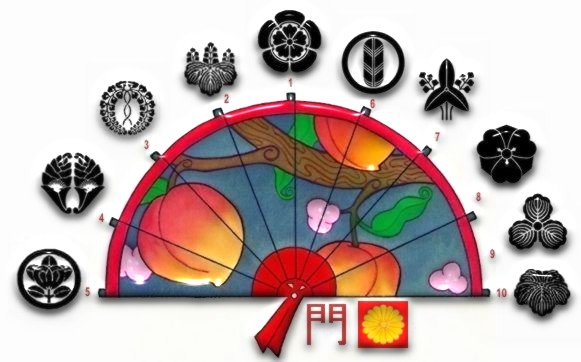This image features a digital interpretation of an East Asian-style fan, resembling stained glass, set against a plain white background with a prominent Photoshop drop shadow. The fan is semicircular with a red border and center, and it showcases a vibrant depiction of a tree branch adorned with peaches, leaves, and delicate pink flowers. The design is segmented by thin black lines, including one that runs vertically down the middle, creating triangular cutouts on either side. 

Numbers from 1 to 10 are labeled along the top, with 1 at the vertical center and increasing outward, flanked by various black plant-like and floral symbols beside each number. These symbols range from different styled flowers to leaves, some within black circles, resembling household crests. At the bottom of the fan, there is a kanji or Chinese character composed of two vertical lines with boxes at the top, separated by a horizontal line. Next to this character sits a red square featuring a yellow, twenty-petaled flower.